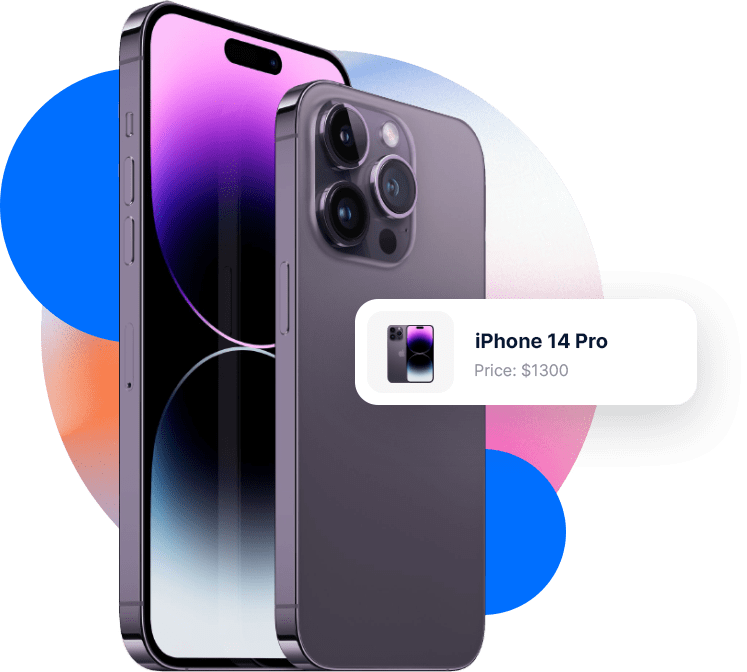This image is a digitally created illustration of an iPhone 14 Pro, tagged with a $1300 price indication. The artwork is not a real photograph but rather a computer-generated graphic. The background is composed of several vibrant circles in hues of blue, purple, orange, pink, gray, white, and other shades. The largest circle is nearly the size of the phone itself, with two smaller blue circles in front but still behind the iPhone.

The iPhone 14 Pro is depicted twice in the image: a larger front-facing view and a slightly smaller back-facing view positioned in front of it. The front-facing illustration displays two or three side buttons, likely for volume and power control. The screen exhibits a mix of colors, including purple, various shades of blue, black, white, and gray. The back view showcases the iPhone's camera setup with two or three lenses accompanied by a flash.